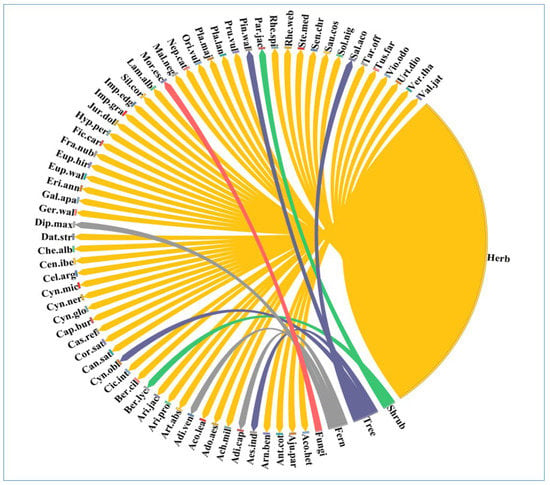The image is a detailed circular chart, predominantly yellow, depicting a variety of scientific names. Surrounding the outer rim of the circle are numerous black-font words, each corresponding to different plant types. Sections within the circle use distinct colors: green for "shrub," blue for "tree," gray for "fern," and red for "fungi," all against a white background. "Herb" is prominently featured on the right side in black text, occupying nearly one-fifth of the circle, where no lines extend from it. Various lines—some straight, some arcs—connect the words on the outer rim to the inner sections of the circle. Phrases like "par jack" and "bear lie" stem from "shrub;" "sal," "ocko," "pin," "wall," and "sin obl" connect to "tree;" "oddy cop," "ocko," "jay," and "dip max" link to "fern;" and "more esky" associates with "fungi." The overlapping colors and detailed labels around the circle suggest a complex categorization, with the yellow portion and the isolated "herb" segment being particularly notable.